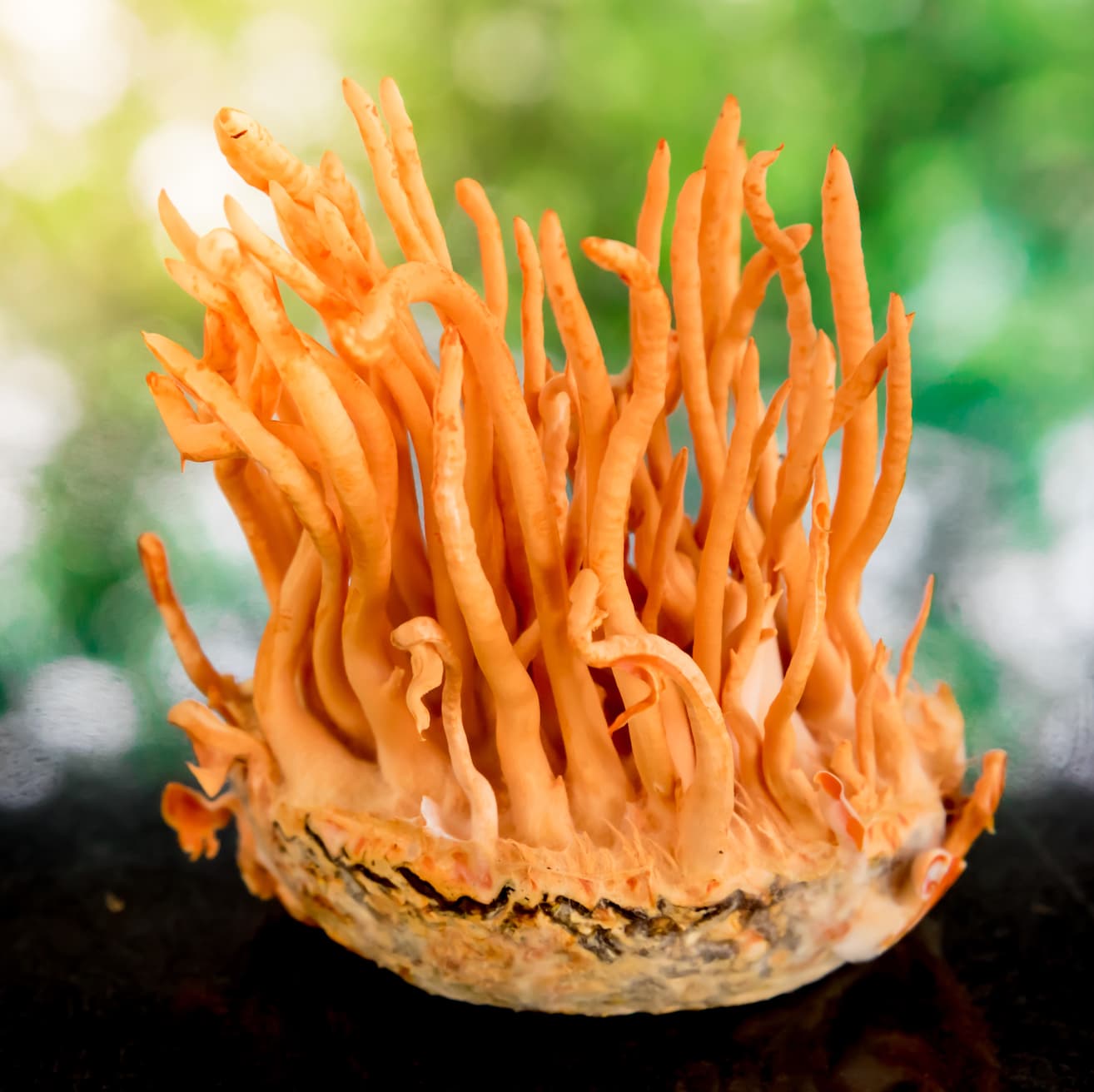The image captures a mysterious orange object, resembling a sculpture but with an organic complexity that's hard to define. The focal point is a central figure, appearing to be a black stone or base, from which numerous orange, coral-like strands or tentacles emerge, radiating upwards in a wavy pattern. The strands exhibit a clay-like texture and create an intricate, unique design. There is speculation that this object could be an exotic sea creature like a sea urchin or sea sponge, or even a type of fungi with a multitude of root-like appendages. The background is out of focus, featuring blurred shades of green and white, perhaps indicating plants with light filtering through, and the base of the image hints at a dark surface that could be dirt or a wooden table. Overall, the image is brightly lit, emphasizing the vibrant orange of the central figure while the indistinct background adds a sense of depth and mystery.